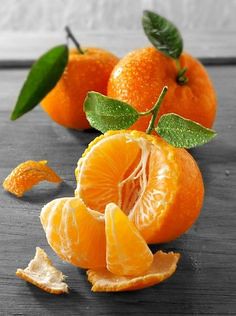The photograph features a trio of vibrant oranges arranged on a light gray wooden surface, likely a table or floor, against a plain white wall. The focal point is the closest orange, which is partially peeled with a few segments detached and resting on the peel itself. This orange stands upright with a small stem adorned with two vivid green leaves. Behind it, two intact oranges retain their shiny, wet-look peels, each with a petite stem and a single leaf. One of these back oranges presents its stem and leaf toward the viewer, while the other shows a larger, prominent green leaf. The arrangement captures the freshness and natural aesthetic of the oranges, with careful attention paid to their stems and leaves, adding a touch of greenery to the composition.